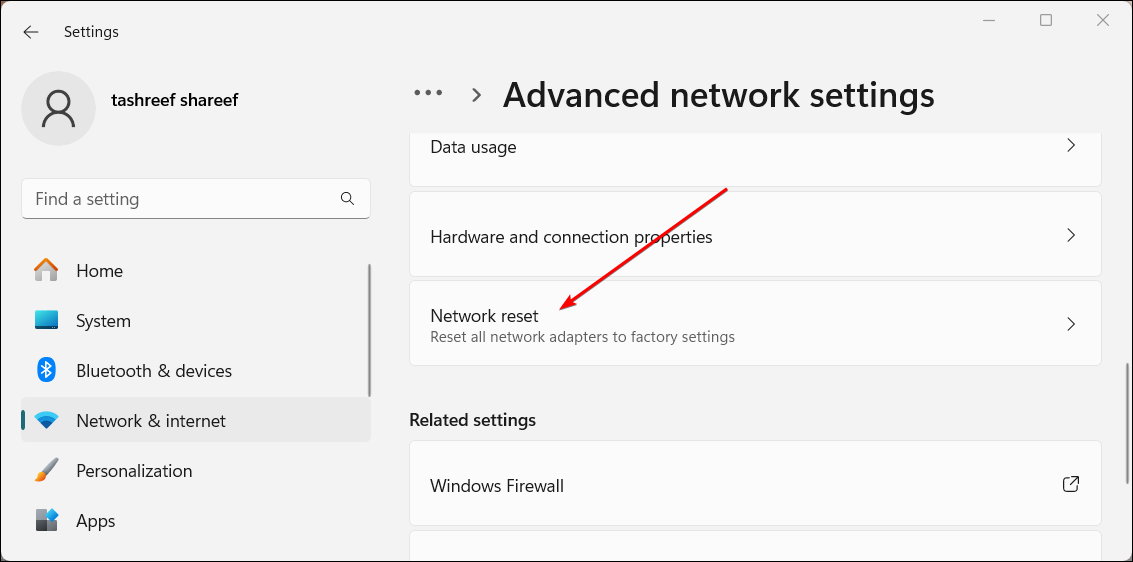In the image, we see an advanced network settings page, likely from a Windows operating system, designed for the user Tashreef Sharif. The interface includes standard window controls—minimize, maximize, and close—in the upper right-hand corner. Below these controls, there is a search bar titled "Find a setting."

On the left-hand side, a navigation menu lists several settings categories, including Home, System, within Devices, Network & Internet, Personalization, and Apps. These categories are organized in a vertical sidebar.

Prominently displayed on the right is the "Advanced Network Settings" section, highlighted with a context menu and an arrow, denoting its importance. Directly below, several options are available: 

1. Data Usage
2. Hardware and Connection Properties
3. Network Reset

A notable detail is a red arrow pointing specifically to the "Network Reset" button, indicating its significance in this context. This image is part of a training guide on how to reset network settings.

Further down, under the "Related Settings" section, "Windows Firewall" is listed. Although the full list isn't visible, it is suggested there might be additional settings accessible by scrolling further.

The overall layout and elements suggest functionality typical of a Windows settings interface, though similar designs can be seen in torrent applications or router settings pages.